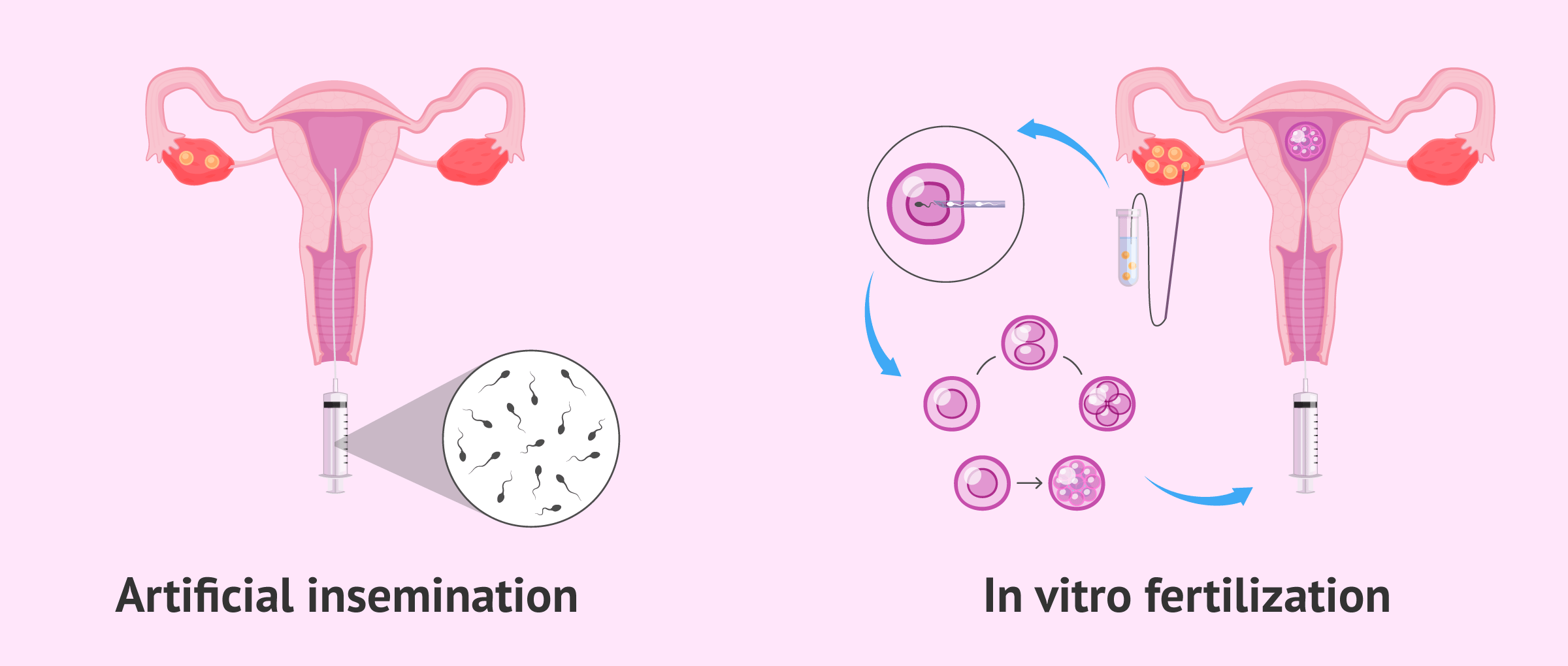The image illustrates and compares the processes of artificial insemination and in vitro fertilization (IVF). It features a light lavender and light pink rectangular background populated with various anatomical diagrams. On the left side, near the bottom, the text "artificial insemination" is displayed. Below this text, there is a depiction of the female reproductive system highlighting the fallopian tubes. In this section, black tadpole-like representations of sperm are shown being introduced into the fallopian tubes to meet the eggs, which appear inside a white circle. 

The "in vitro fertilization" section displays a similar anatomical diagram of the female reproductive system but includes additional blue areas that illustrate the stages of the IVF process. Highlighted within this section is a sequence involving five purple circles, which likely represent the developmental stages of eggs. The colors used throughout the image include white, gray, purple, pink, orange, and black, which are primarily used for text and anatomical details. The image effectively demonstrates the flow and different steps involved in these two reproductive technologies.